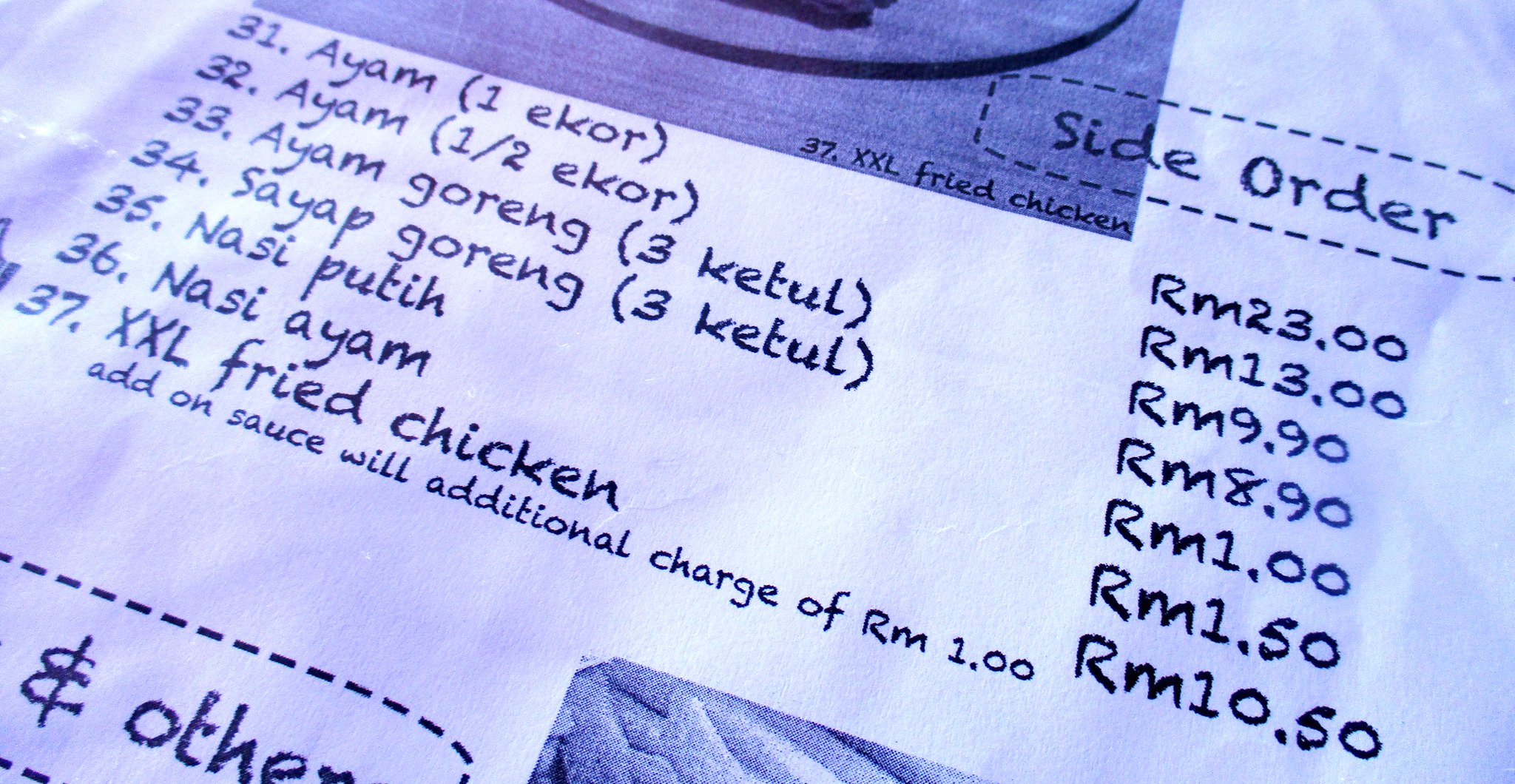The image depicts a menu from what appears to be either an Indian or Chinese restaurant, but most likely features Malaysian dishes given the items listed. The menu is predominantly blue with white background. In the upper center, there's a darker blue area with some text, and specifically, in the lower right corner, it says "Fried Chicken."

The top right corner of the menu highlights a section called "Side Order" in blue, within a rectangular dotted area. Underneath this section, various menu items are listed:

- 31. Ayam (1 Ekor) - RM 23.00
- 32. Ayam (1/2 Ekor) - RM 13.00
- 33. Ayam Goreng (3 Ketul) - RM 9.90
- 34. Sayap Goreng (3 Ketul) - RM 8.90
- 35. Nasi Putih - RM 1.00
- 36. Nasi Ayam - RM 1.50
- 37. XXL Fried Chicken - RM 10.50

An additional note mentions that adding sauce will incur an extra charge of RM 1.00. At the bottom part of the menu, there's partial text reading "other" in blue, and to the right, a small image resembling breadsticks can be seen against a light blue background.